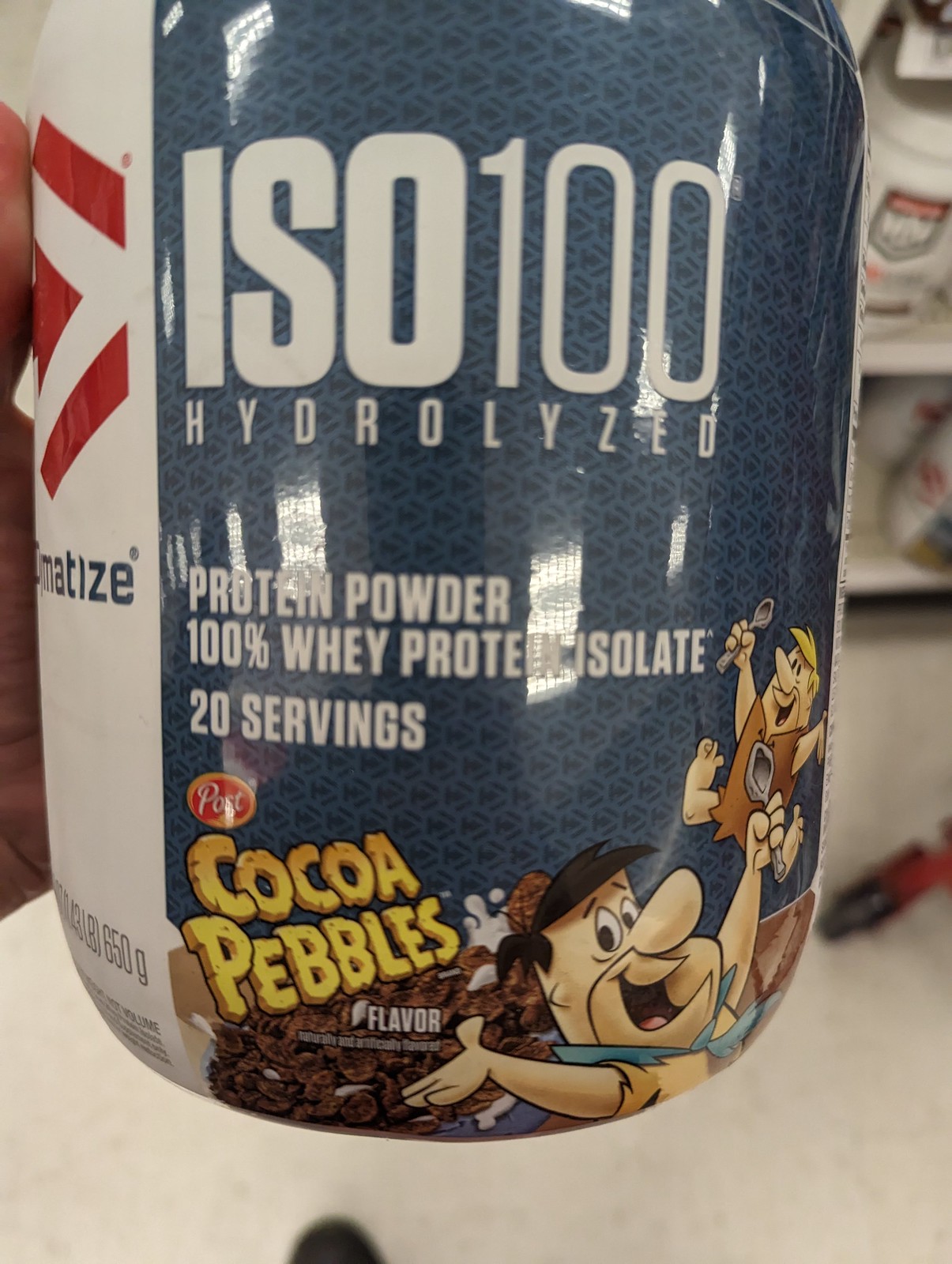This is a digitized, color photograph showcasing a 650-gram container of ISO 100 hydrolyzed protein powder, prominently featuring the Cocoa Pebbles flavor branding. The container predominantly displays blue and white colors with red accents. Toward the bottom of the container, the iconic Fred Flintstone and Barney Rubble characters from "The Flintstones" are joyfully holding spoons, celebrating the Cocoa Pebbles flavor. They are positioned above a bowl filled with Cocoa Pebbles cereal and splashes of milk. The label on the plastic-coated jar reads "ISO 100 Hydrolyzed Protein Powder, 100% Whey Protein Isolate, 20 servings." Reflections of large window panes can be seen on the bottle’s shiny surface. The bottle appears to be floating against a blurred white background, which includes indistinct shelves and a pen, and is held by a barely visible hand on the left side of the image.